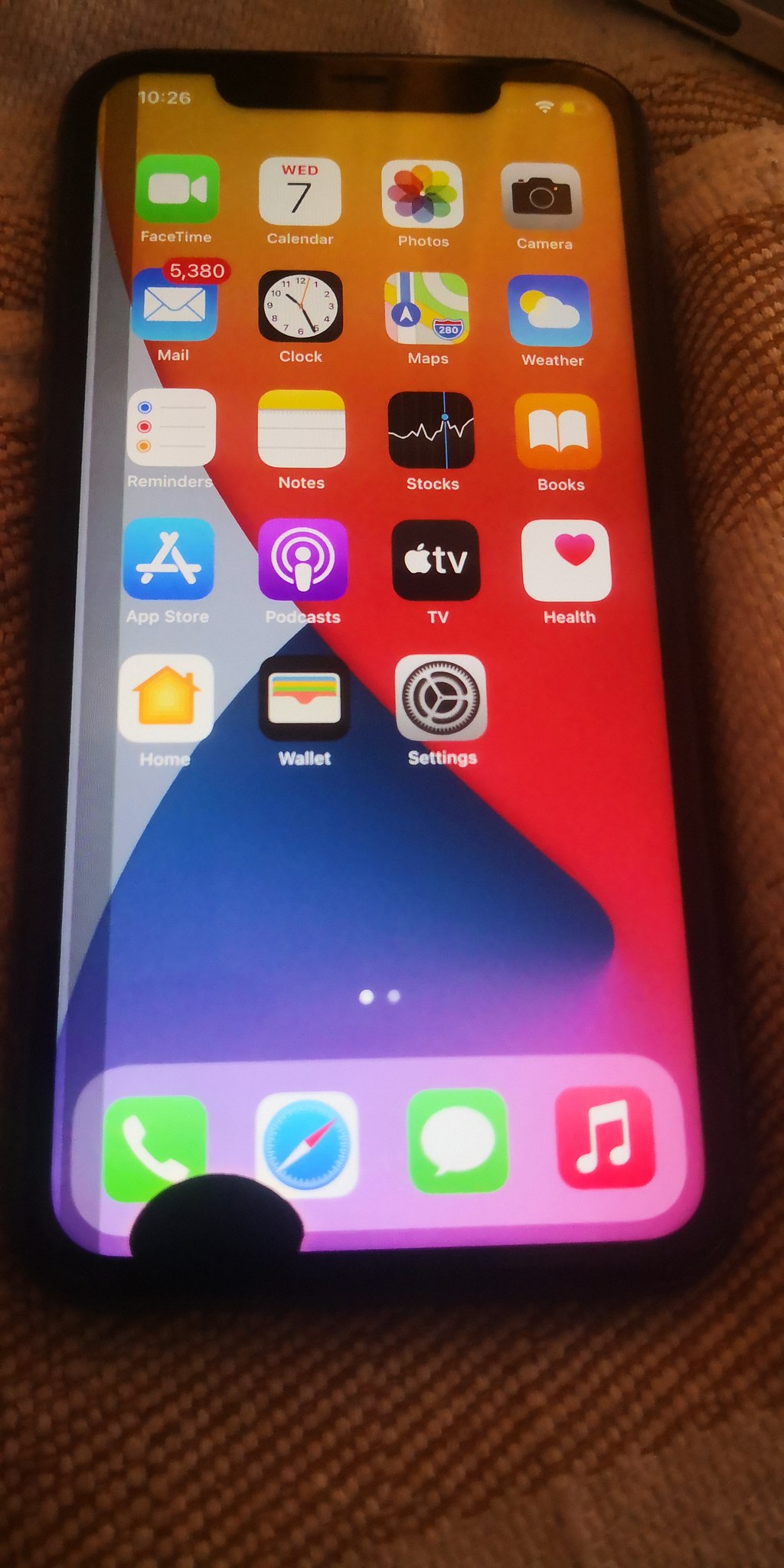This vertical photograph captures a smartphone lying atop a vibrant orange woven plaid blanket. The phone's screen is lit up, displaying the current time as 10:26 in the upper left corner. The screen is outlined by a black border and includes a variety of app icons arranged in a grid pattern. Along the bottom of the screen, there are specific icons for phone, location, messaging, and music functionalities. The phone's background showcases a dynamic mix of geometric shapes in orange, red, blue, and white hues, transitioning to a purple shade at the bottom. A dark arched shadow is visible at the lower left corner of the screen, while another shadow runs down the entire left side. The phone also indicates a strong Wi-Fi connection, a half-filled battery icon, and two small white dots situated at the very bottom of the display.